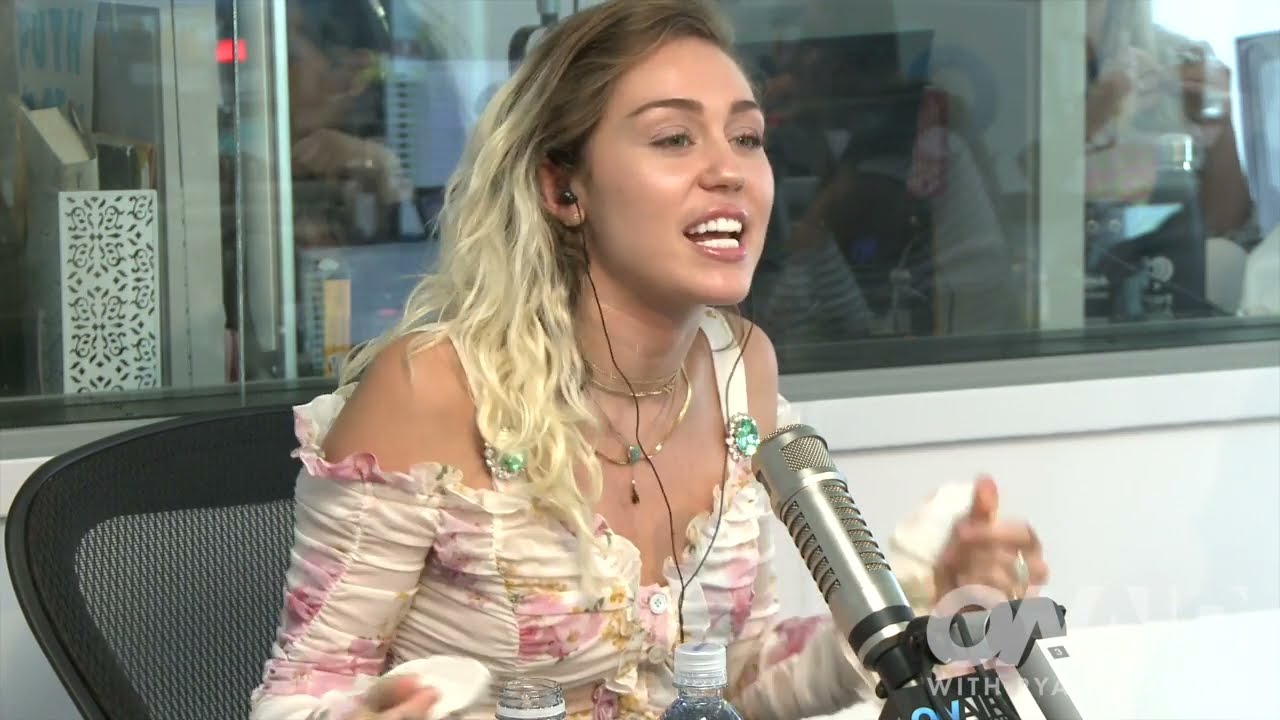Miley Cyrus is captured mid-interview at a radio station, seated in a black chair behind a white desk. She is wearing a white floral dress adorned with pink and lavender flowers, featuring off-shoulder white straps adorned with green brooches surrounded by diamonds. Her wavy, bleached blonde hair cascades slightly below her shoulders. Miley is engaged in conversation, leaning forward with an open mouth, revealing her teeth and a cheerful demeanor. She has earbuds in her ears with a visible dangling cord. A gold necklace with a tiny green charm adorns her neck. Her hands are slightly blurred in motion, indicative of her animated speaking style. The thick, silver microphone in front of her contrasts with the clean white desk. Behind her, large glass windows reveal an adjacent room with blurred offices and onlookers, adding depth to the scene. Miley's minimal makeup highlights her clean complexion, complementing her overall vibrant and engaged presence.